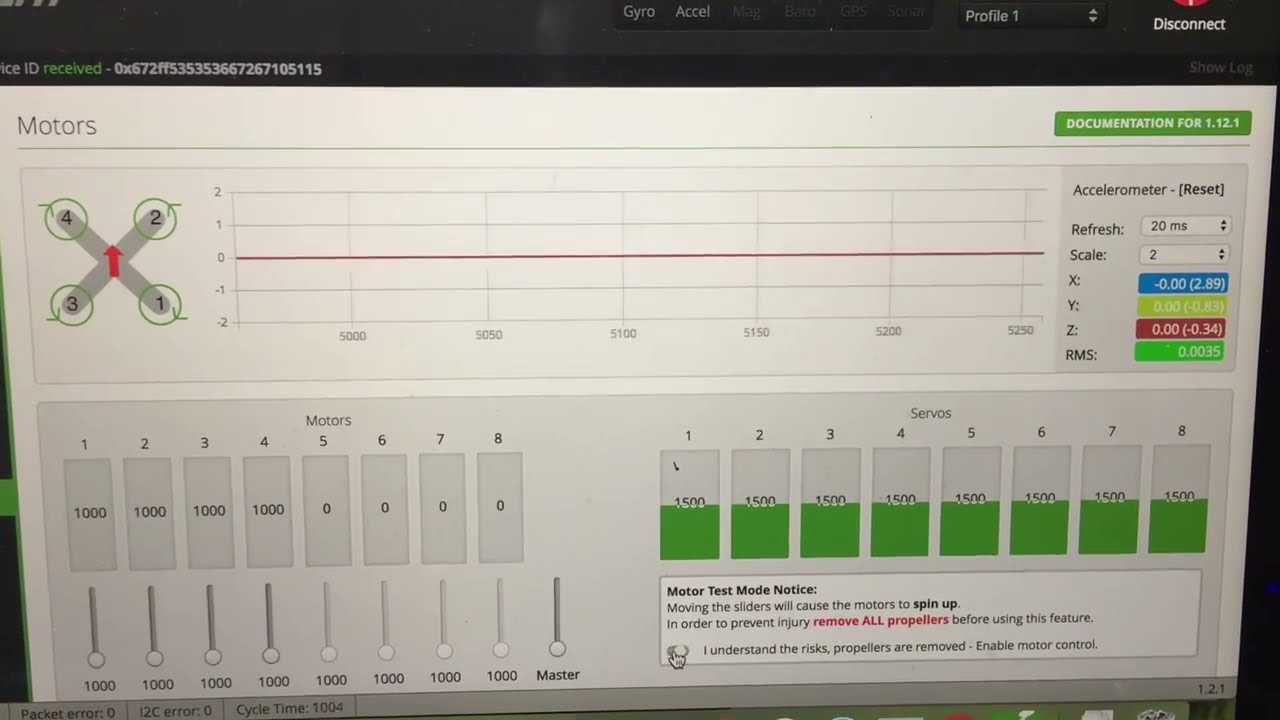The image depicts a computer screen monitor displaying a user interface (UI) that is predominantly white with gray boxes. The UI is focused on motor testing and information. In the upper left corner, there is an identifier labeled "ID received" in green, followed by a series of white numbers "0X672FF535353667267105115." The upper right corner features a black bar with the word "disconnect," and beneath it is a green tab labeled "documentation for 1.12.1."

Central to the UI, a gray box labeled "accelerometer reset" is prominently displayed. The left column contains four colored boxes with numerical data and the label "refresh scale XYZRMS." 

A significant area on the bottom displays various sliders, all set to 1000, and next to them is a white box with black font stating "Motor Test Mode Notice." The notice warns in black text that "moving the sliders will cause motors to spin up," and emphasizes in red text, "remove all propellers," before continuing in black text with "before using this feature." Additionally, there is a checkbox that reads, "I understand the risk, propellers are removed, enable motor control." 

The lower part of the screen also features several gray tabs, with some tabs on the right side highlighted in green at the bottom. This detailed interface is part of what seems to be a motor testing setup, ensuring user safety through clear instructions and warnings.